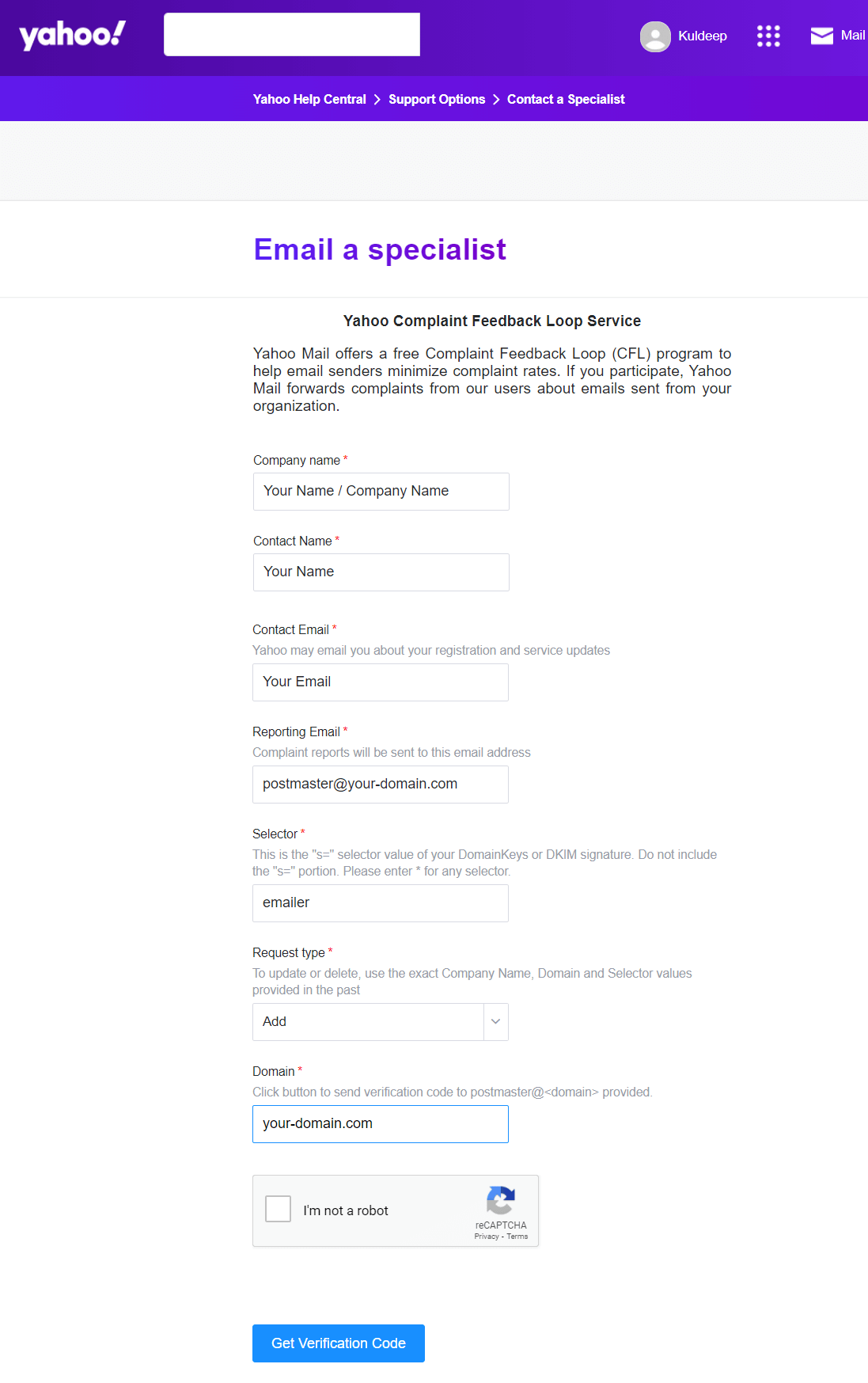A screenshot from the Yahoo website is displayed with a purple border at the top. The Yahoo logo, featuring "Yahoo!" in white print, is prominently positioned on the left. Adjacent to the logo is a white search bar. In the upper right corner, there is a gray profile icon labeled "Call Deep," accompanied by a letter icon for mail. Below these icons, white print reads: "Yahoo Help Central, Support Options, Contact a Specialist."

Further down, on a white background, a bold purple heading states: "Email a Specialist." In black font underneath, it spells out: "Yahoo Complaint Feedback Loop Service. Yahoo Mail offers a free Complaint Feedback Loop (CFL) program to help email senders minimize complaint rates. If you participate, Yahoo Mail forwards complaints from its users about emails sent from your organization."

The page then continues with several form fields to register for the service:
- **Company Name**: Your name/company name
- **Contact Name**: Your name
- **Contact Email**: Your email
- **Reporting Email**: postmaster@yourdomain.com
- **Selector**: emailer
- **Request Type**: (shown as a drop-down menu labeled "Add")
- **Domain**: your-domain.com

At the bottom, there is a checkbox for "I am not a robot" verification, accompanied by a Recaptcha challenge. An interactive blue button labeled "Get Verification Code" is also present, indicating functionality for form submission.